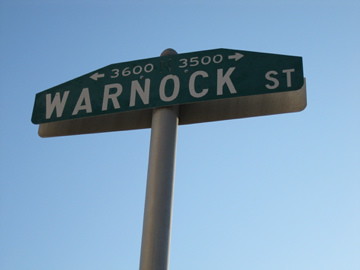In this clear and vibrant photograph, we see a single green street sign mounted on a metal pole against a strikingly blue sky. The sign, which dominates the image, features large white text that reads "Warnock ST" with "ST" abbreviated and smaller. Above "Warnock," to the left, the sign depicts an arrow pointing left with the number 3600, while an arrow pointing right with the number 3500 is on the right. The sign itself is rectangular but has a distinctive triangular peak at the top. In the background, the sky transitions from light to a slightly darker blue as you move from the bottom to the top of the image, accentuating the sign's presence. Another sign can be slightly seen behind it, likely providing similar directional information for the opposite direction.